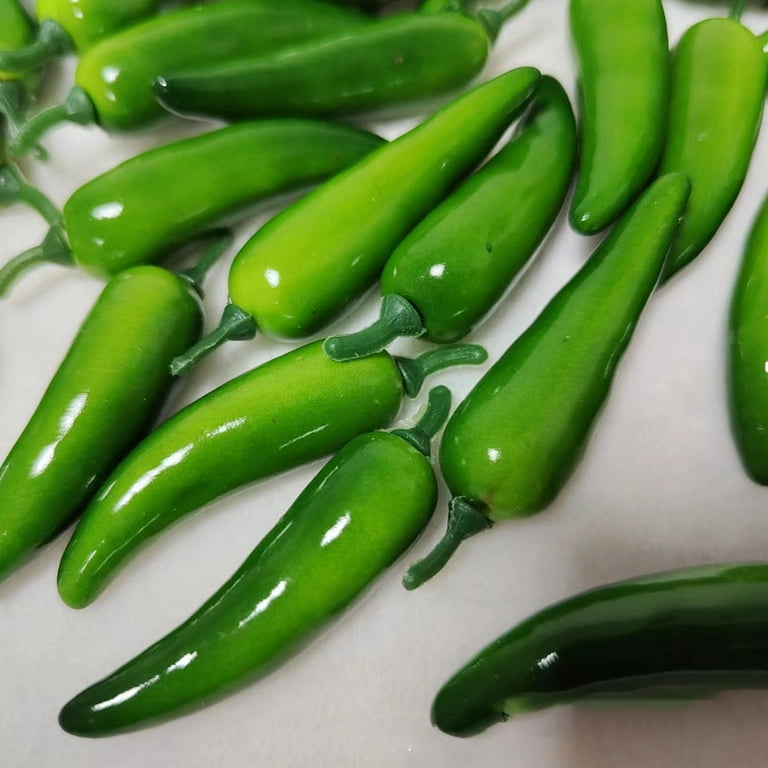The detailed photograph showcases a scattering of approximately a dozen green jalapeno peppers arranged loosely on an off-white surface. The vibrant, medium-green peppers are exceptionally shiny and smooth, each one featuring a dark, curved stem. Despite their realistic appearance, upon closer inspection, it becomes evident that they are artificial, made entirely of plastic. The peppers are well-lit, with a noticeable glare of light enhancing their glossy finish. The image, resembling a realistic photo or perhaps AI-generated, is closely cropped, focusing solely on the peppers without any surrounding elements such as people, animals, or text. The softness and slight blur of the peppers further from the camera contribute to the natural, yet deceptive, initial impression of authenticity.